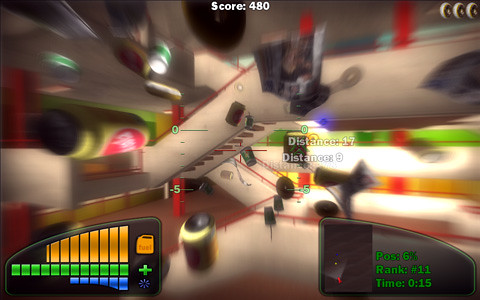This image is a detailed screenshot from a video game, showcasing various in-game annotations and the navigational space the player is exploring. At the top of the image, the word "Score: 480" is prominently displayed in white font, indicating the player's current score. 

At the bottom, a dial resembling a vehicle's fuel gauge is visible. The gauge has an icon of a fuel can, together with a series of bars colored green, amber, and blue, signifying the fuel levels. Adjacent to the fuel gauge, another window provides crucial player metrics, including "Position: 6%", "Rank: 11", and "Time: 0.15".

The main body of the screenshot reveals a complex, three-dimensional environment that the player is navigating. It features multiple flights of stairs arranged in a labyrinthine manner, suggesting various levels and pathways to explore. The scene is vividly colored with reds and yellows, enhancing the immersive experience. This screenshot captures the intricate design and detailed statistics of the game, highlighting the player's progress through this multi-level, visually vibrant environment.